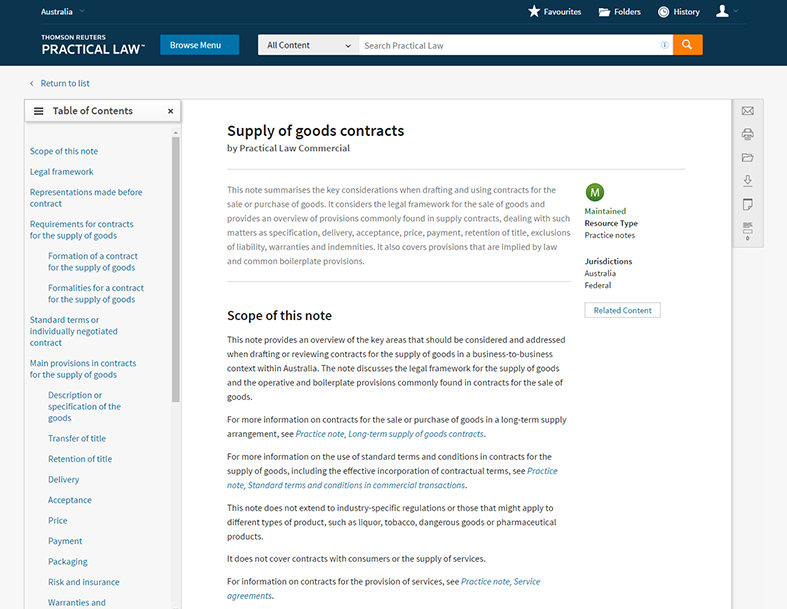The header of the webpage features a prominent blue button labeled "Australia," accompanied by the "Thomson Reuters Practical Law" logo below it. Adjacent to this, a blue button titled "Browse Menu" is positioned. To its right, a dropdown bar marked "All Content" is followed by a search box with an orange button bearing a magnifying glass icon. Above this search section, navigation options include "Favorites," "Folders," and "History," alongside a small person outline symbol representing the user profile.

Beneath these elements, a blue-text "Return to List" option with a left-pointing arrow sits atop the main content area. Here, a box labeled "Table of Contents" contains several lines of blue text. The focal point of the page is a detailed description titled "Supply of Goods Contracts" by Practical Law Commercial, followed by an explanatory paragraph. Adjacent to this paragraph is a green circle with a white checkmark, indicating the content is "Maintained."

Further details specifying "Resource Type," "Practice Notes," and "Jurisdiction: Australia, Federal" are listed below in black text. A white button with blue text labeled "Related Content" is also available. To the left, another text section begins with the header "Scope of This Note," presenting multiple explanatory paragraphs about the legal concept.

At the top right of the page, just below the main blue header, small icons for email, print, save, and download functionalities are accessible for user convenience.